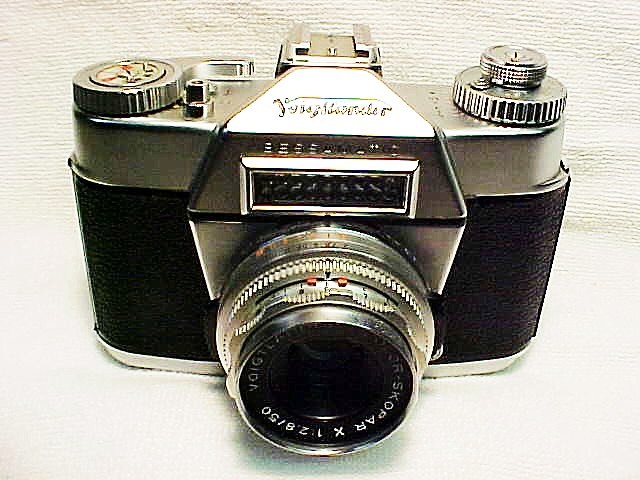This image captures a vintage black and silver analog camera set against a white background with a line pattern resembling tissue paper. The centerpiece is a protruding lens encased in multiple layers of metal, with inscriptions reading "128150" and "S-K-O-P-A-R" around its edge. Flanking the top of the camera are two silver dials—one on the right and one on the left—designed to adjust various settings. The brand or model name is inscribed at the top center, though it is not clearly legible in the image. Additional details include a small button near the left dial, likely used for advancing the film or taking pictures.